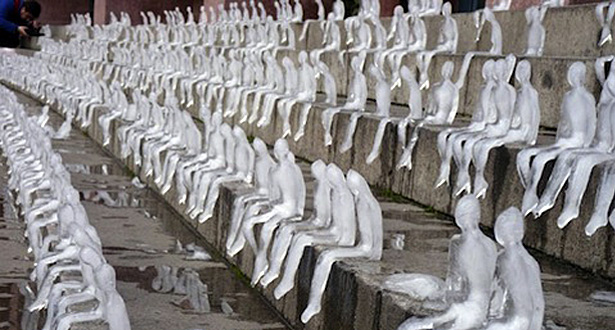This image presents a compelling digital artwork that merges photography and painting. The scene features a series of slightly curved cement or stone steps resembling simple stadium seating or an amphitheater. On these steps, rainwater has collected in puddles, and darker streaks, possibly from moss or water runoff, mar the vertical surfaces. The primary artistic addition is the array of ghostly white silhouettes of people, who appear to be standing or sitting on the edges of each step, filling the entirety of the steps much like a crowded stadium during an event. These figurines lack any detailed features such as faces or clothing, giving them a spectral, ice-like appearance. The interplay of the physical steps and the painted figures creates an eerie, yet captivating, visual experience. Additionally, in the upper left corner of the photograph, there is a barely visible person crouching, possibly with a camera, seemingly capturing the scene, adding a layer of intrigue and mystery to the overall composition.